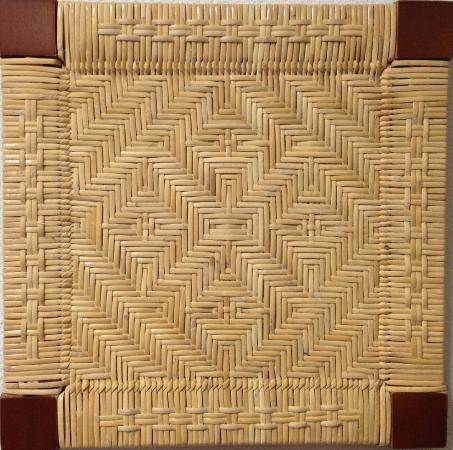The image features a tan-colored box-like texture adorned with a series of intricate patterns. At the center of the image lies a square shape, which is embellished with a diamond-shaped design in its very middle. Surrounding this central diamond are four additional smaller diamond shapes. Each of these shapes is defined by intersecting diagonal lines, also in the tan color, creating a cohesive and intricate design. Encircling the central square are four rectangular shapes: vertical rectangles on the left and right sides, and horizontal rectangles on the top and bottom. The corners of the image are marked by a rich brown color, forming square-shaped backgrounds in all four corners, which contrast with the predominantly tan hues, further emphasizing the central design.